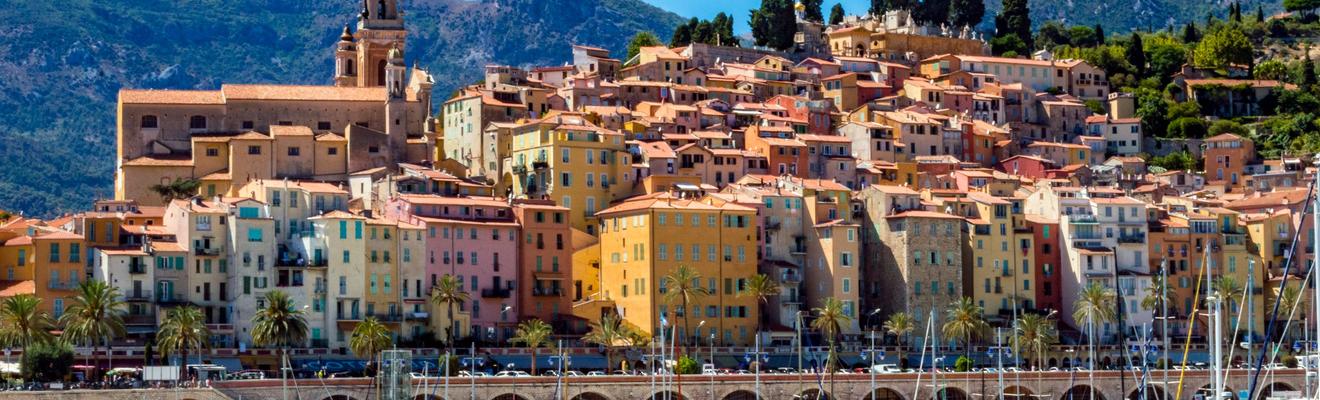The image depicts a vibrant coastal city stretched along a waterfront, viewed from a fair distance over the water. The cityscape features numerous apartment buildings closely stacked against each other, adorned in a palette of pastel shades including pink, yellow, beige, orange, red, and brown. These buildings gracefully ascend a hill that culminates in a green, tree-studded mountain in the background.

At the foot of the city, adjacent to the water, a long bridge is lined with palm trees and sparse smaller trees, creating a picturesque promenade where people can be seen walking. The marina in the foreground is dotted with small sailboats and boats, emphasizing the city's strong boating or fishing culture. Alongside the marina, several vehicles are parked, and a fence runs parallel to the water, adding to the urban atmosphere.

The entire setting basks under a bright blue sky on a sunny day, further enhancing the idyllic and warm coastal environment of this lively and colorful town.